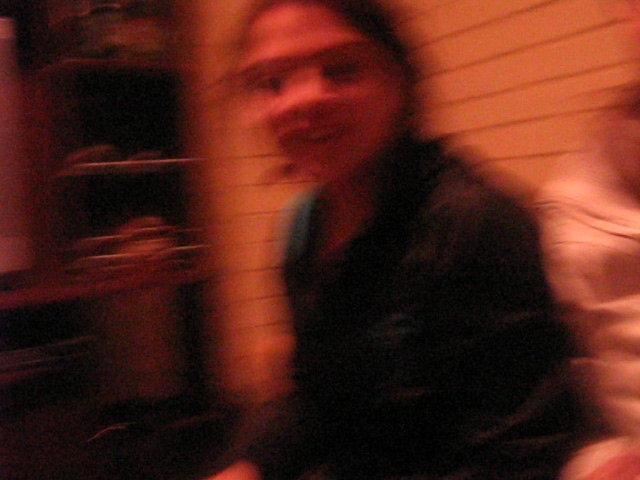The blurry photograph features a person who appears to be female, characterized by an indistinct visage with black hair and dark eyes. The pixelation gives an illusion of a unibrow and an unusually wide nose, while their eyes seem notably wide-set. Although the image suggests a smile, it is likely a result of motion blur either from the camera or the subject moving. The individual is wearing a black, long-sleeved polo shirt. Next to them, there seems to be another person in white. The background includes a white brick wall, with a brown bookshelf to the left. The bookshelf has multiple shelves, each containing indistinguishable items.